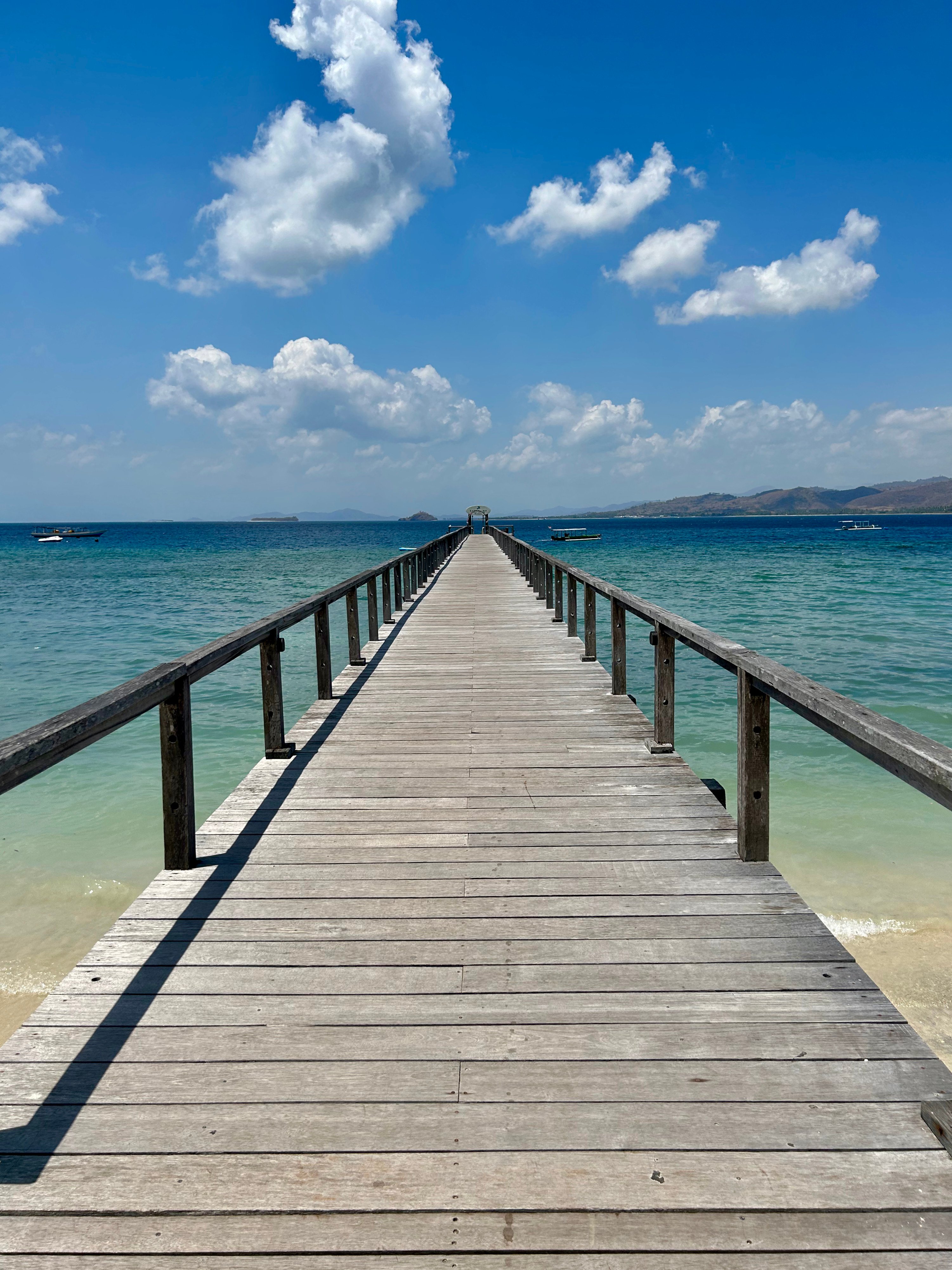This vibrant photograph captures a picturesque pier extending into the ocean from the vantage point at the shore. The pier, constructed of aged yet sturdy gray wooden planks with handrails on both sides, stretches out to a distant, barely discernible structure at its end. The scene is bathed in natural light under a brilliant blue sky punctuated by puffy white clouds. The ocean water transitions beautifully from a light clear hue near the sandy shore to a deep blue out in the distance, where small whitecaps are visible. To the sides of the pier, the sparkling blue ocean stretches out, dotted with several sailboats, one notably to the left and a couple more to the right. Along the distant horizon, the shoreline continues with lush green hills rolling down to meet the water, and the faint silhouette of another town or mountainous area blends with the sky, adding to the breathtaking view. No people or animals are present in this serene capture.